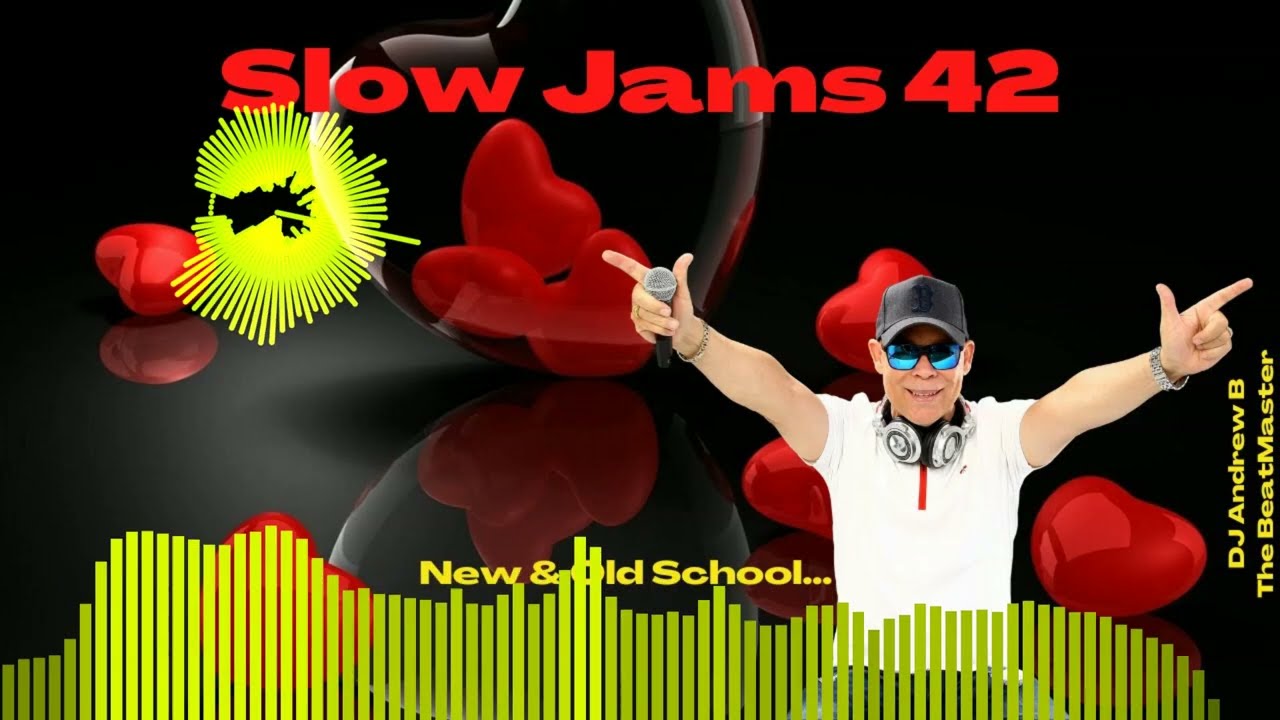The image features a promotional advertisement for "Slow Jams 42" rendered in vibrant colors and graphics. Dominating the black background are patterned green hearts, alongside 3D-like clear hearts with red centers. At the top of the image, "Slow James 42" is prominently printed in red text. An older gentleman, presumably DJ Andrew B. The Beatmaster, stands near the right side of the visual. He dons a sporty, white short-sleeved t-shirt with red accents around the collar, blue reflective sunglasses, and a black cap. Two bracelets, or perhaps a bracelet and a watch, adorn his wrists. Over-the-head earphones dangle on the back of one leg. He strikes a dynamic pose with both arms extended forward and upwards, pointing, and holding a microphone in his right hand. Below him, running across the bottom of the image, are striking yellow and lime green lines resembling sound waves. Adding to the vintage-modern theme, the words "New and Old School" are displayed centrally at the bottom. To his right, in conjunction with more text, the phrase "DJ Andrew B. The Beatmaster" is integrated into the design. The overall aesthetic combines elements of red, green, yellow, blue, tan, silver, and gold, making for a visually engaging announcement for this musical event.